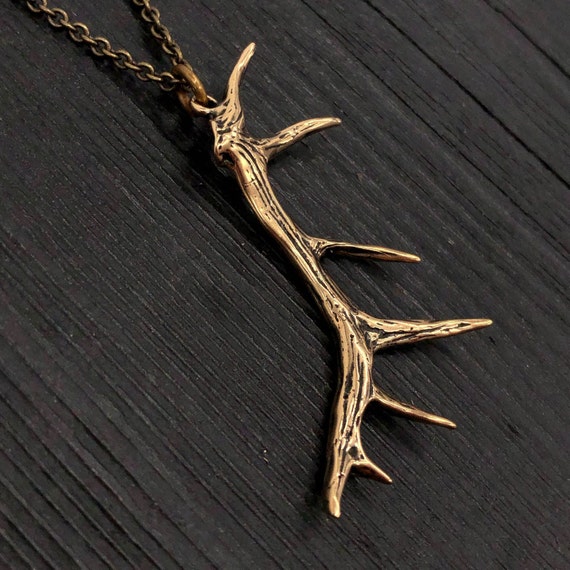The photograph showcases an intricate piece of jewelry featuring a twig-like ornament made of metal, possibly copper, bronze, or brass, finished with a dark patina to give it an aged appearance. The branch ornament is adorned with multiple offshoots, resembling thorns, and exhibits natural striations filled with a blackened patina, highlighting the fine details. This rustic ornament is suspended from a delicate chain, also made of a similarly darkened metal. The necklace is meticulously displayed on a black-tinted wooden surface, with subtle wood grain lines adding texture and creating a stark, contrasting backdrop that enhances the visual focus on the piece. The overall composition suggests a carefully crafted, perhaps artisanal, style, making it a likely product for an online boutique or an Etsy shop.